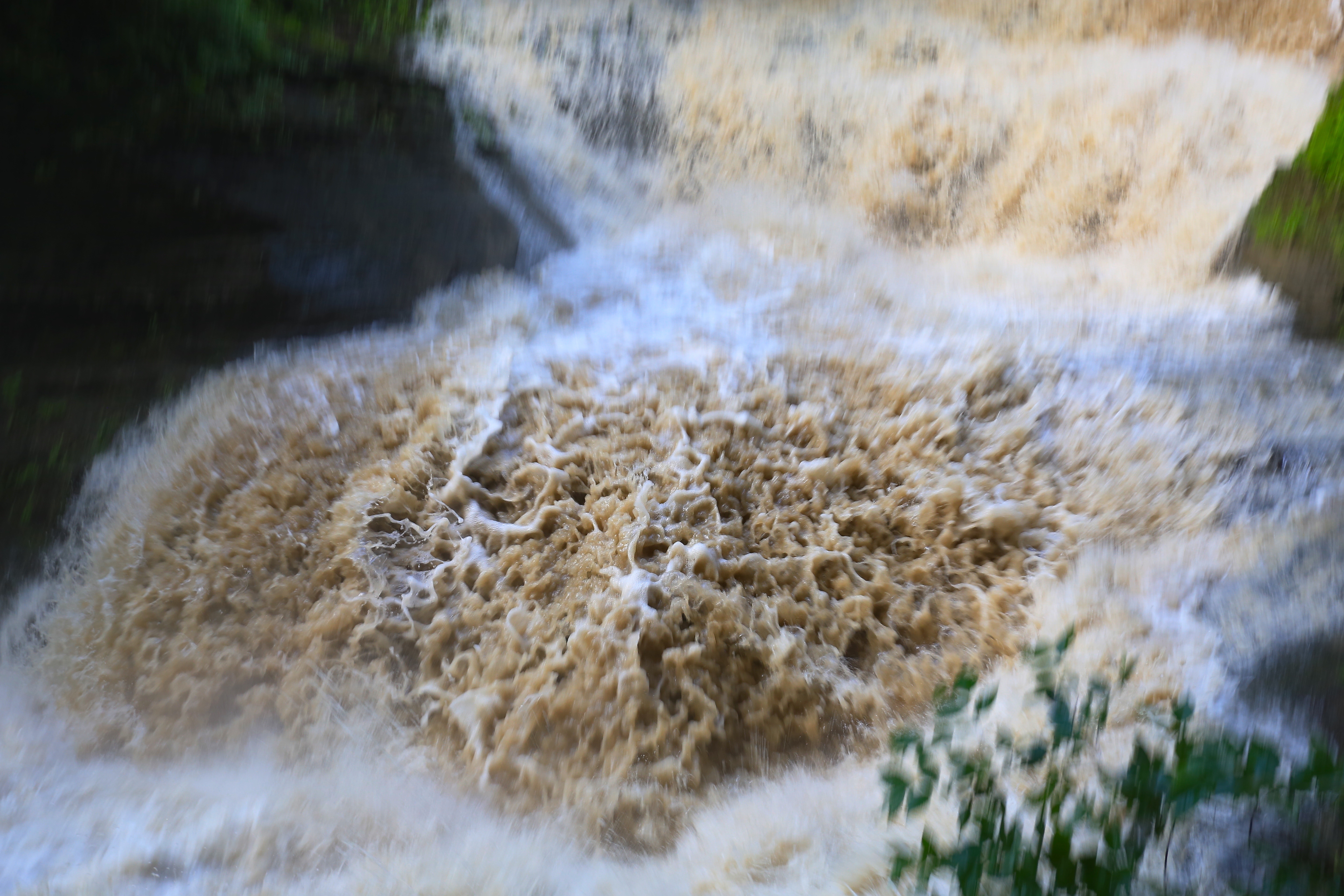The photograph captures a dynamic outdoor scene, centering around a turbulent, foamy rush of water. In the midsection, the water appears murky with a mix of brown hues, suggesting a high content of sediment and dirt, while it peaks and froths, creating a highly textured look. In the background, although slightly out of focus, there seems to be a waterfall with water cascading down, highlighted by white foam and interspersed with yellowish-brown patches. The foreground features a partially blurred bush or tree, displaying green leaves and thin branches. The top left corner of the image contains a mysterious black area, possibly part of a mountain or an undefined shadow.